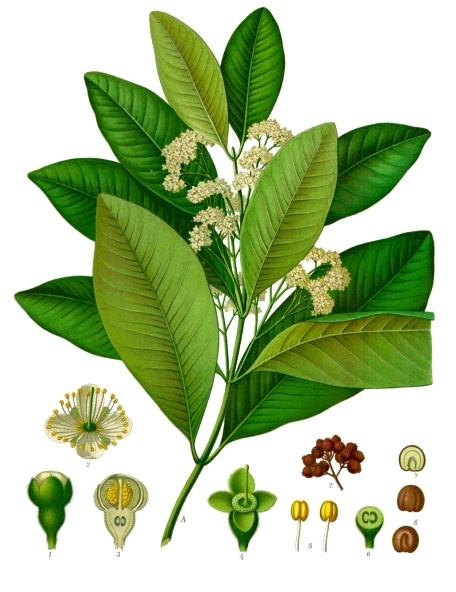This detailed illustration features a green plant with a long central stem adorned by leaves of varying shades of green. There are approximately seven darker green leaves and four lighter ones, which might be the undersides. The leaves are large, narrow, and pointed, with a rounded shape along the sides. Clustered around the center of the plant are tiny, delicate white flowers resembling baby's breath.

At the bottom part of the illustration, there are several detailed images of different parts and stages of the plant, labeled for scientific clarity. On the left side, a series of three images display a green bud, an open flower, and a close-up of the white flower. On the right side, additional illustrations include a four-leaved green plant, two yellowish buds, a green section, a red berry-like structure, and three vertically aligned seeds or nuts, each with distinct colors and markings. The entire composition appears to be meticulously drawn, likely using various colors of ink, set against a white background for a clear and detailed botanical presentation.